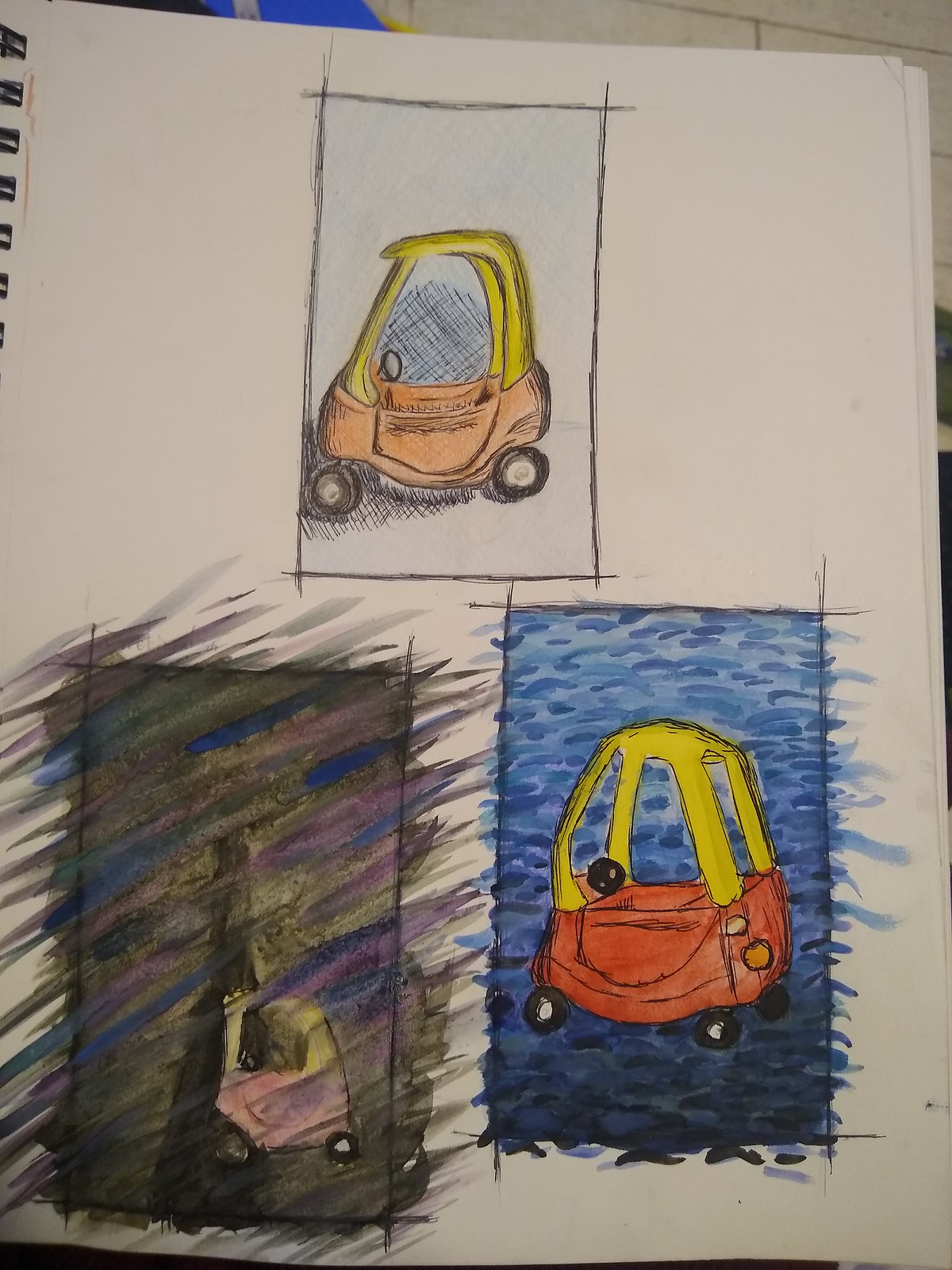This image features a tiled wall in the background, providing a textured yet neutral setting. In the foreground, there is a spiral-bound sketch pad, opened to a page on the right side. The top portion of the page displays a vertical rectangle with a light blue background, showcasing a child's ride-on toy car. The toy car is designed with a yellow roof, a red body, and black wheels, indicative of a play car that children can sit in and drive around. On the lower right of the page, the same image of the car is recreated against a black background, this time illustrated with markers, giving it a contrasting, bold appearance. To the left of this depiction, a similar image of the toy car is overlaid with erratic, jagged black lines, creating a scribbled effect that conveys a sense of deliberate defacement or a chaotic artistic expression.